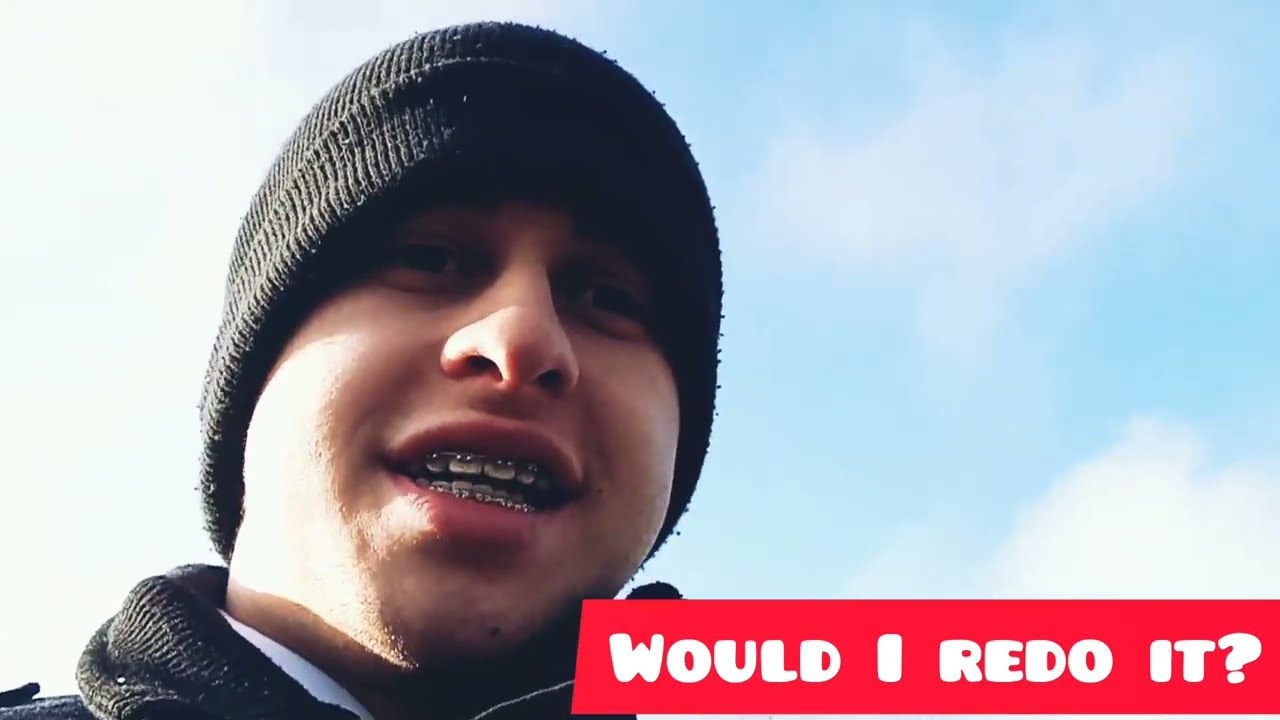The photograph features a young man, likely in his late teens or early twenties, with braces on his teeth. He has light skin and a bit of baby fat on his face, indicating a youthful appearance. He is wearing a black knitted beanie that is pulled down over his eyebrows, casting a shadow that obscures his eyes. He is dressed in a black jacket with a thick collar, suggesting it is a cold day.

The image is taken from a low angle, making it appear that the man is looking down towards the camera. The sky in the background is a mix of blue with patches of white clouds. The man takes up the left portion of the image, while in the bottom right corner, there is a red horizontal box with white text that reads, "Would I Redo It?" The man appears to be either talking or simply has his mouth open, displaying his tightly wound braces. The context of the text remains a mystery, adding an element of intrigue to the photograph.